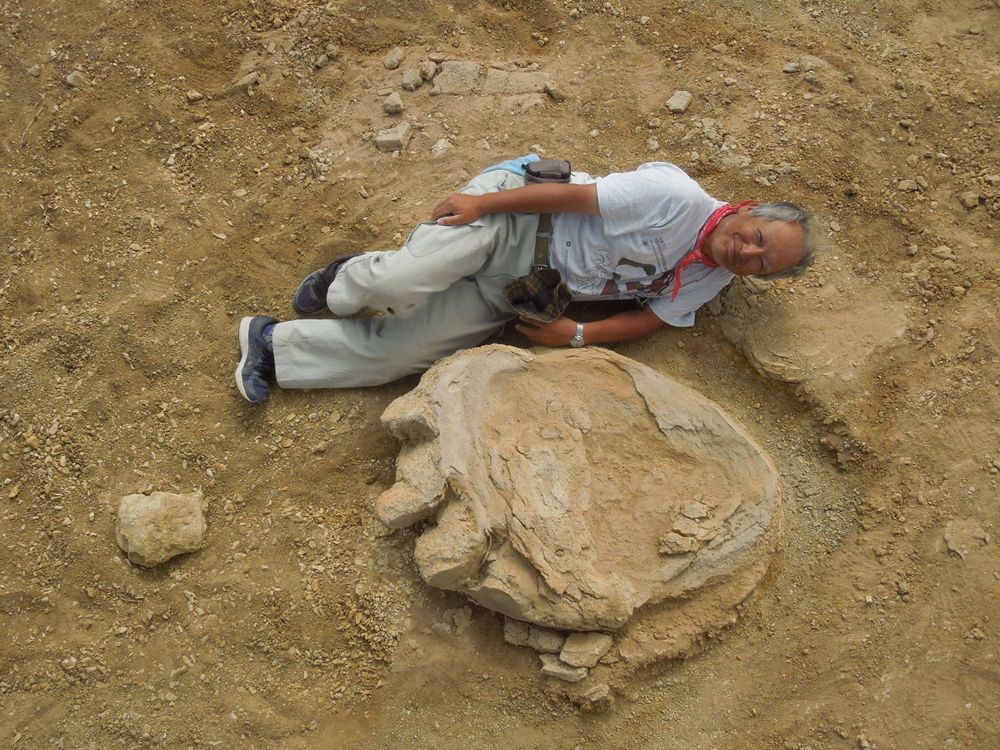The photograph shows a man lying on light brown dirt next to a large, foot-shaped fossil. The man, who appears to be older with grayed hair and possibly of Asian descent, is positioned above the fossil in the frame, gazing up at the camera, which captures the scene from an overhead perspective. He is wearing black shoes with white soles, khaki-colored cargo shorts, and a brown belt with a pouch on one side. His outfit is completed with a short-sleeved gray shirt (partially hidden by folds), and a distinctive red and white bandana tied around his neck. The fossil, which resembles a large, clawed foot with a pattern suggesting a possible dinosaur origin, is surrounded by fragmented rocks and sandy terrain, adding to the sense of an archaeological or paleontological discovery.